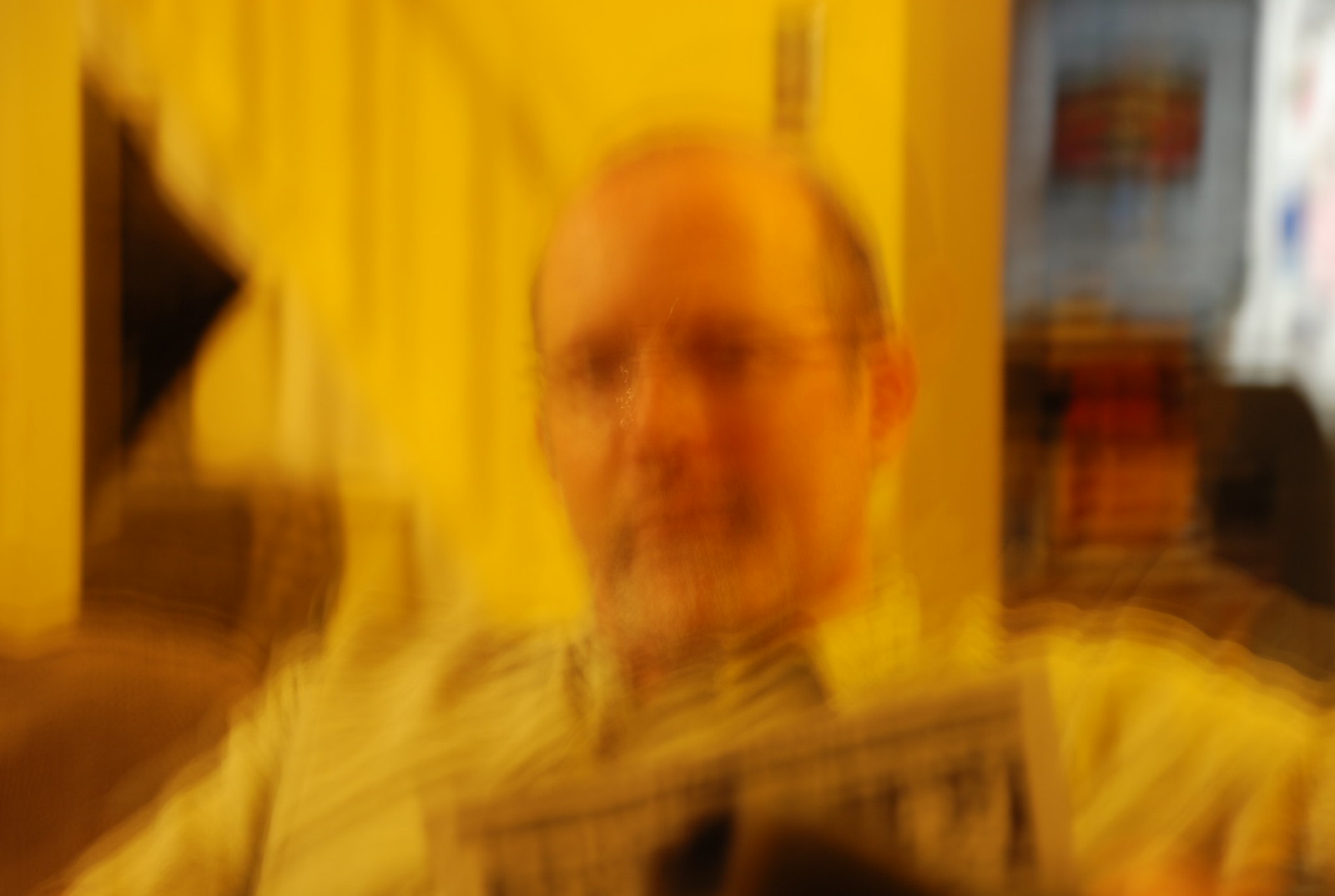In this extremely blurry photograph, a man is seated on a brown couch, visible from the chest up. The overall lighting of the scene has a yellowish hue, which may contribute to the appearance of his shirt being yellow, though it could also be a white-collared shirt. The man is balding with hair on the sides above his ears and is wearing thin, wire-framed glasses. He has a beard and mustache and appears to be holding a magazine, with just the top of it visible. He looks directly at the camera, his facial features including dark-colored eyes and a closed mouth are discernible despite the blurriness. 

In the background, on the left side, there is a brown, almost circular staircase against a yellow wall, and on the right side, a glimpse into another room with a blue wall. Details in this adjacent room include a painting, a large brown piece of furniture, and possibly a brightly lit window with white curtains. The entire image remains indistinct, giving an overall hazy view of the scene.